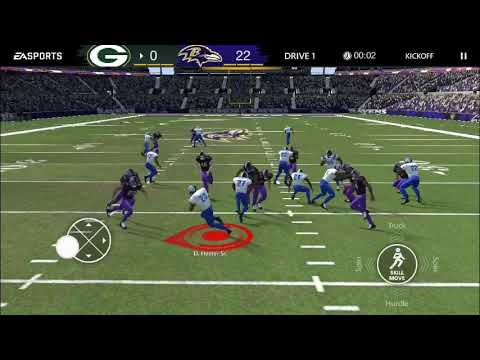This widescreen screenshot, complete with black bars on the top and bottom, captures a mid-play moment in an American football video game, reflected through its detailed UI. The top black bar prominently features the EA Sports logo, followed by the scoreboard displaying a Green Bay Packers logo with a score of 0, and a Baltimore Ravens logo with a score of 22, indicating that the Ravens are leading. The display also shows the drive information, noting it's the first drive with a kickoff occurring, and just 2 seconds remaining on the timer. The scene is set in a typical stadium filled with spectators, showcasing a long view from one side of the field. Players from the Green Bay Packers are wearing purple and white uniforms, while the Baltimore Ravens players sport purple and black attire. The realistic in-game rendering immerses the viewer in a competitive match, highlighting the intricacies of the digital realm of EA Sports' football game.